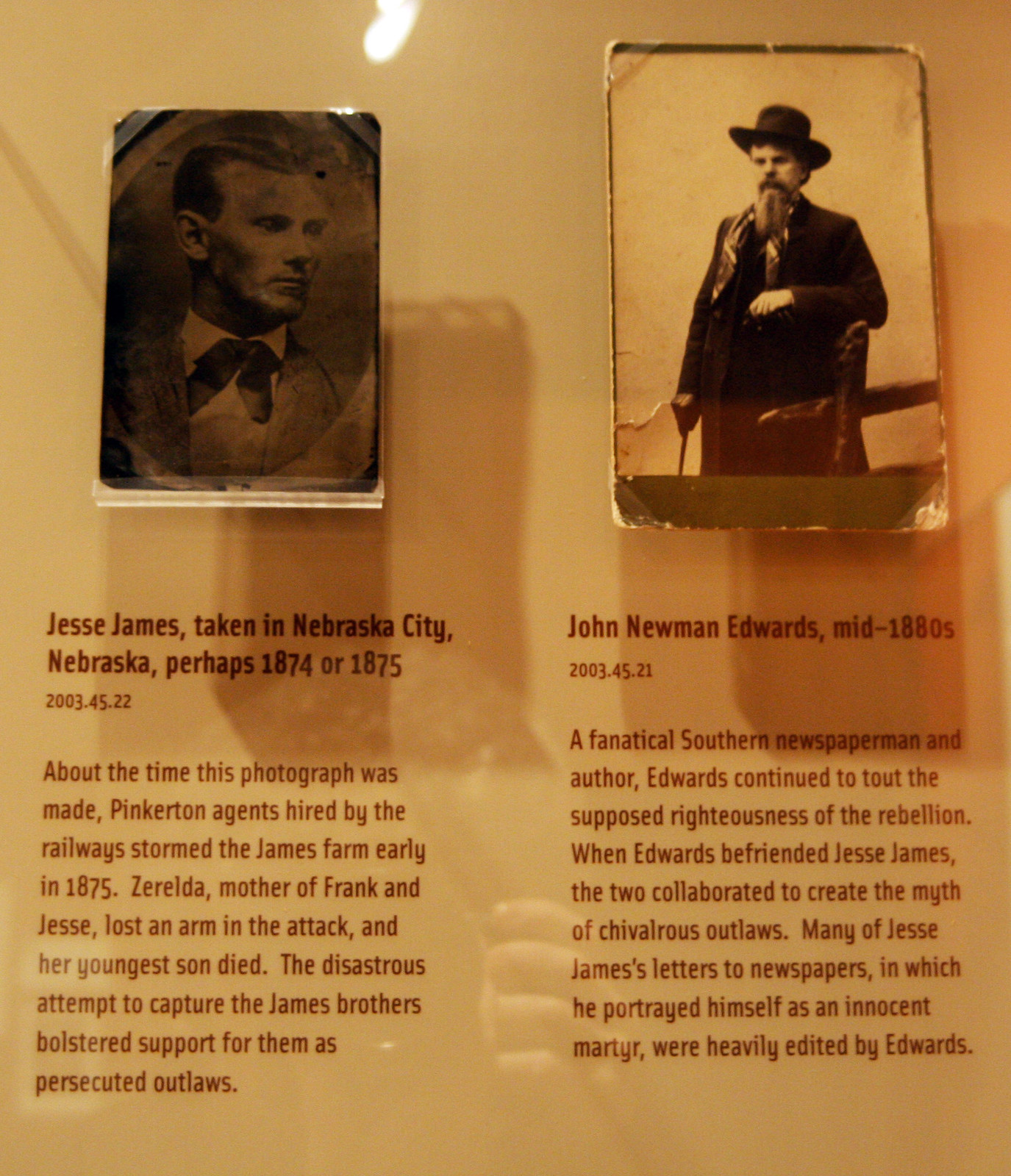The image showcases two century-old vintage black and white photographs on a glossy, reflective surface, with text descriptions below each. The first photograph on the left features the infamous Jesse James, captured in Nebraska City, Nebraska, around 1874 or 1875. The detailed caption notes, "Jesse James taken in Nebraska City, Nebraska, perhaps 1874, 1875." A paragraph beneath elaborates on a significant event from that era, indicating that in early 1875, Pinkerton agents hired by the railways stormed the James farm. Jesse's mother, Zerelda, lost an arm in the attack, and her youngest son died, an event that ultimately garnered increased support for the James brothers, casting them as persecuted outlaws. The photograph of Jesse James, though deteriorated, shows him dressed in a suit, gazing to the right.

The second photograph on the right depicts John Newman Edwards, a fervent southern newspaperman and author from the mid-1880s. The caption reads, "John Newman Edwards, mid-1880s," and details his role in romanticizing Jesse James through media. Edwards befriended James and together they crafted a narrative of chivalrous rebellion. Many of Jesse James' letters to newspapers, portraying himself as an innocent martyr, were heavily edited by Edwards. The image shows Edwards in a dark, large coat, holding a stick in one hand, with a beard and a large round cap, and one arm resting in front of his chest.

Overall, the image not only presents historical portraits of Jesse James and John Newman Edwards but also delves into their intertwined legacy, highlighting their collaboration in shaping the mythos of the American outlaw.